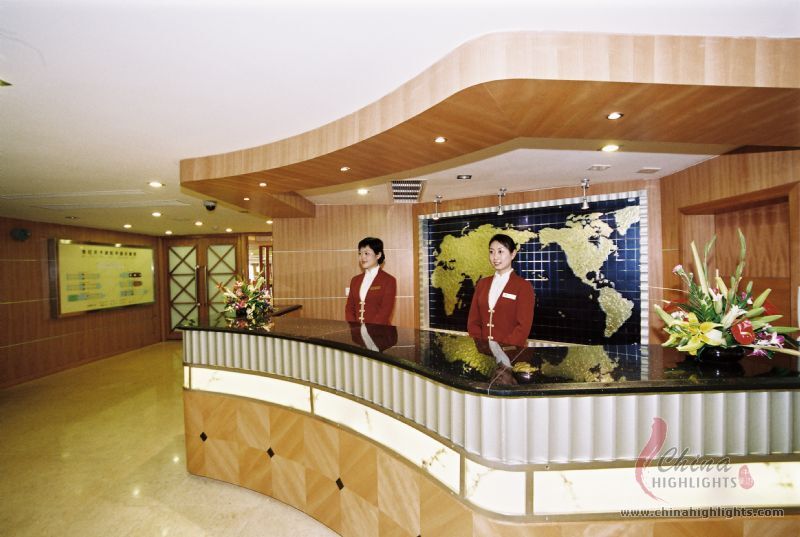In the image, a hotel lobby's front desk is manned by two individuals in red jackets with off-white dress shirts underneath. They stand directly in the center of the image, partially obscuring a blue and yellow map of the world that forms the backdrop. Both individuals, who appear to be Asian, have black hair; one with short hair and the other with longer locks. Although they are wearing name tags, the names are not discernible. The desk they are standing behind has a glossy black counter, supported by a section featuring medium to light brown squares and tan tiles. Flanking the desk are arrangements of flowers, adding a touch of elegance amidst the polished tile floor. The ceiling above mirrors the desk with a white surface and brown accents. To the bottom right of the image, the text "China Highlights" is visible along with the website "www.chinahighlights.com". Additionally, a doorway and a hanging sign are seen on the left side of the image, signifying the indoor hotel setting.